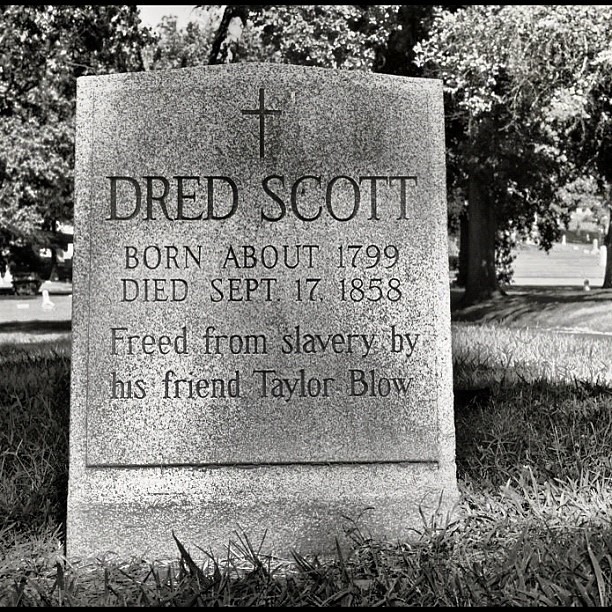This detailed black-and-white photograph captures a solemn scene in a cemetery, focusing closely on a single, worn gray tombstone surrounded by long grass. The headstone prominently features a cross at the top, with the inscription: "Dred Scott, born about 1799, died September 17, 1858, freed from slavery by his friend Taylor Blow." The refined sunlight casts subtle shadows across the image, adding texture and depth. In the background, tall trees with their branches and leaves frame the cemetery, where a few other headstones can be faintly observed in the distant right side of the horizon, contributing to the peaceful yet historic ambience.